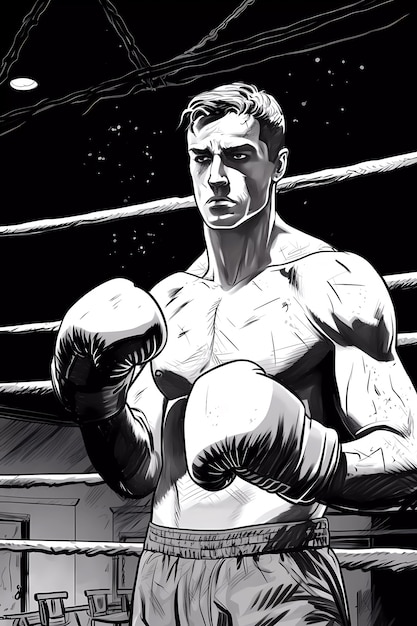This black and white illustration depicts a muscular, shirtless boxer with a stern expression and dark, reflective eyes. Rendered in a graphic comic book style, the drawing is rich in shadows and dimensions. The boxer, possibly modeled after Rocky Balboa, stands in a fighting stance with his gloved fists raised. He wears elastic-waisted pants, resembling basketball shorts. The background features the ropes of a boxing ring and outlines of empty chairs and tables, suggesting a setting inside an arena. The upper part of the image intriguingly blends a dimly lit ceiling with light scaffolding and stars, creating an atmospheric contrast between the immediate indoor environment and the celestial night sky above.